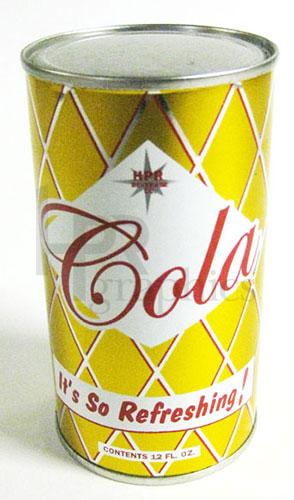The image is a close-up, indoor color photograph of an old, unopened cola can set against a stark white background, casting a faint gray shadow to the left. The can, which appears to be from the 1940s or early 1950s, is predominantly bright yellow with a distinct criss-cross design that forms diamond shapes, reminiscent of a metal cage or fence but purely decorative. At the center of the can, a large white diamond features the word "cola" in red script, topped by a silver star. Below, a smaller white rectangular banner in red font reads, "It's so refreshing!" This is followed by the text, "Contents 12 FL OZ," indicating the amount in fluid ounces. The can, likely made of steel rather than modern aluminum, has a smooth top that would require a can opener, lacking the contemporary pull-tab design. There's also a watermark overlaid on the image, hinting at its vintage nature. Additionally, a logo that reads "HPR Brewing" can be seen at the top middle of the central diamond.